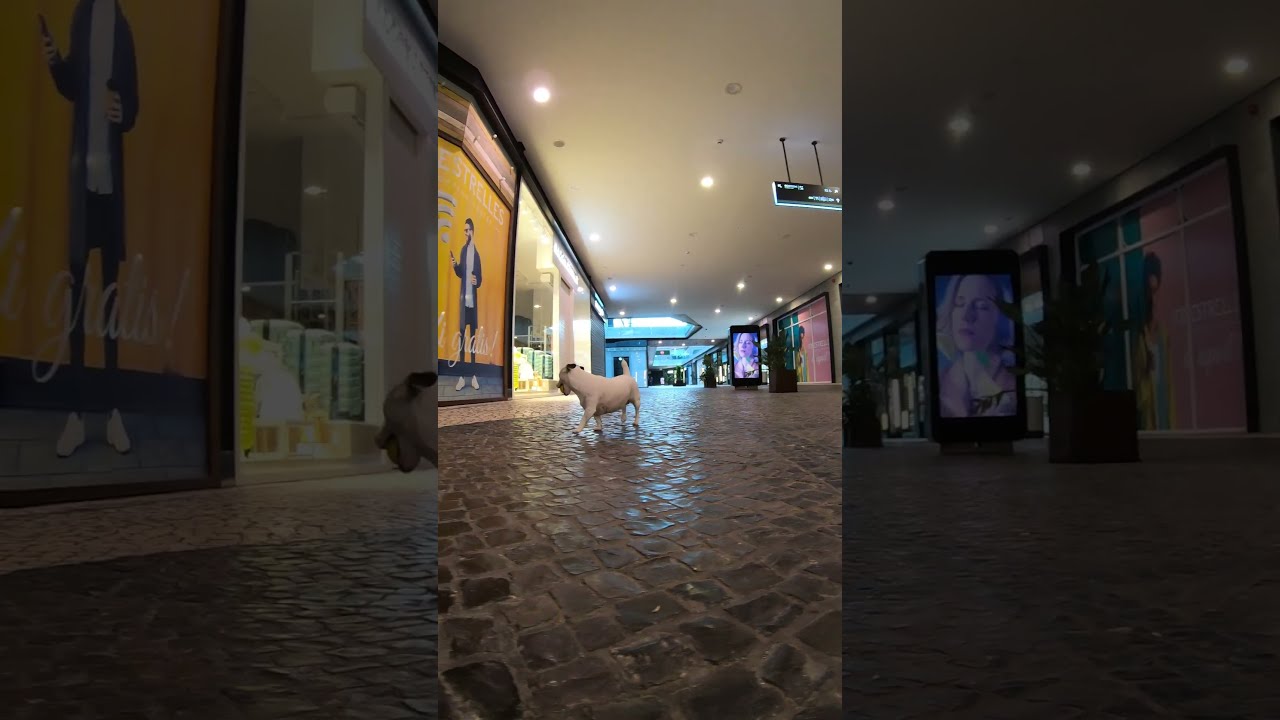In the image, a small, white Jack Russell Terrier with a brown head and short legs walks alone in the center of a shopping mall or indoor plaza. The floor features a cobblestone pattern in brown and gray hues, adding a rustic charm to the otherwise modern space. Overhead, the ceiling is outfitted with numerous lights, giving the area a well-lit, welcoming ambiance. 

To the left of the dog, a sign features an image of a man looking at his phone with the text "Strelitz" or something similar. Nearby are several yellow posters displaying fashion advertisements. On the right side of the hallway, another sign showcases a woman's face with her eyes closed, flanked by indoor plants—one positioned closer, the other farther away. Farther down the hallway, the mall appears to open up into a darker area, suggesting an entrance or a deeper section of the mall. Despite the vibrant setting with various advertisements and decor, the little dog is the only visible being, giving the scene a peculiar, almost serene isolation.